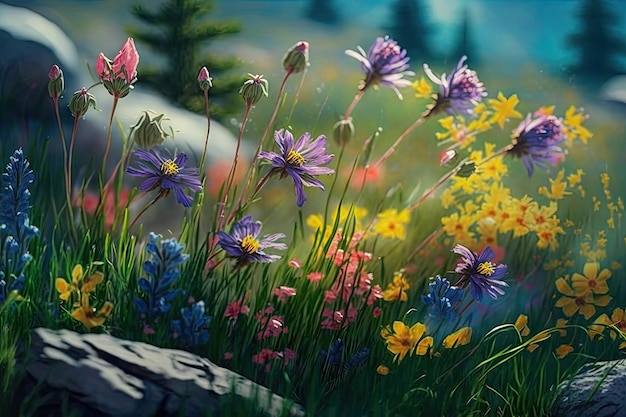This landscape-oriented, AI-generated image captures an up-close view of a diverse array of wildflowers, gracefully illuminated by the soft, warm evening sun. In the foreground, various species of flowers are nestled low to the ground among wild, tall green grass. Vibrant yellow flowers, possibly buttercups with orange centers, stand out prominently. They are accompanied by wild-looking tall purple flowers with yellow centers, tall blue hyacinths with elongated petals, and small, dainty pink flowers, some yet to bloom with tiny pink tips peeking out. The greenery is interspersed with sunlit rocks, grounding the scene in natural beauty. The background of the image is beautifully blurred, suggesting a serene mountainous meadow scattered with large rocks and blurry pine trees, with the ground gently sloping to the right. The sunlight casts a picturesque interplay of light and shadows, completing this stunning depiction of a wildflower sanctuary.